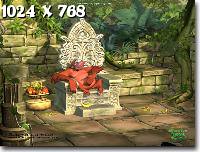This small, digital image, likely a game screenshot, captures the intricate scene of an ancient, potentially Aztec or Mayan-style ruin. The resolution indicated is 1024 x 768, though the image itself is quite small. The structure features a broken, tan brick wall overtaken by jungle vines and greenery, indicative of an abandoned civilization. At the center, a white, intricately carved throne stands, flanked by a bag or pot to the left. Seated on the throne is a striking, red creature, possibly a demon, ogre, or goblin, with elongated arms and a potential tail. Red patio tiles form the floor beneath the throne, leading into the dense jungle backdrop. The bottom right corner of the image contains unreadable text.